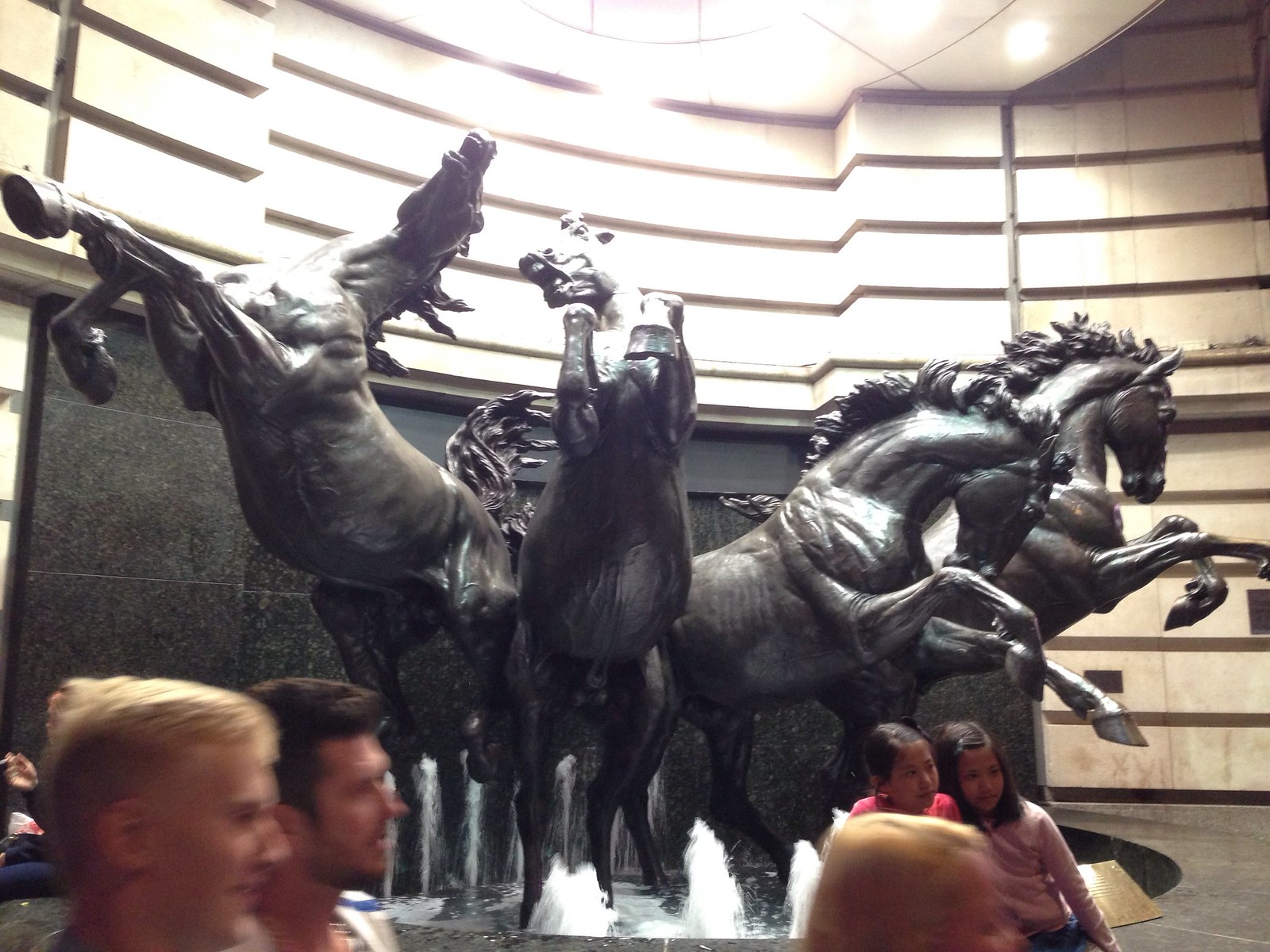In the photograph, set in an elegant indoor environment—possibly a museum or auditorium—a striking fountain takes center stage. This fountain features an intricate statue composed of four large black horses. The horses, crafted from a material that glimmers with tiny white speckles, are depicted in dynamic, rearing poses, each with legs lifted and heads held high or turned in different directions, adding a sense of motion and drama. Their tails and manes flow gracefully, emphasizing their powerful forms. The horses' rear ends are positioned close together, radiating outward in a semicircle, creating a cohesive and captivating centerpiece.

Surrounding the fountain's base, water splashes gently, adding a lively contrast to the solid structure. In front of the statue, two young girls, appearing to be about 10 years old, sit at the fountain's edge, posing for a picture with smiles on their faces. Behind them, three adults—two men on the left and one woman on the right—stand slightly out of focus in the foreground, seemingly distracted by something outside the frame.

The background of the statue is composed of sleek black marble, which is elegantly offset by a section of tan stone slates positioned above it, suggesting an upscale setting. The overall composition of the photograph captures the grandeur and detail of the horse sculpture, while also highlighting the human element with the children and adults engaging in the scene.